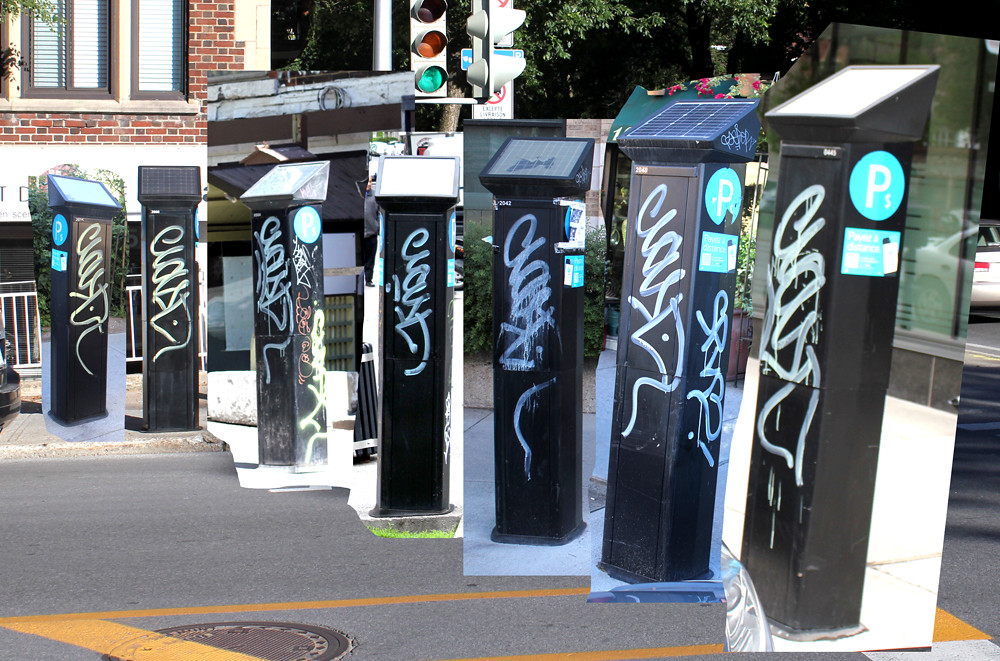This image presents a suburban street intersection, notably enhanced by seven superimposed photos of vertical, solar-powered kiosks. The scene features a horizontally extending street with traffic lines, a traffic light situated behind the center kiosk, lush trees, and a red-and-white brick building with brown-framed windows on the left side. A silver or gray car is parked off to the middle right.

The kiosks, arranged in a diagonal line from the top left to the bottom right, appear prominently in the foreground. Each kiosk is tall, black, topped with a solar panel, and bears identical graffiti tags of the word "Claude" in white spray paint. Additionally, each kiosk displays a teal logo featuring a white "P" with a smaller dollar sign to its right, and an obscure sticker underneath that resembles the words "pair" and "distance."

The integration of these kiosks into the street scene underscores an element of visual juxtaposition, as the spliced images of the kiosks starkly contrast with the serene suburban background.